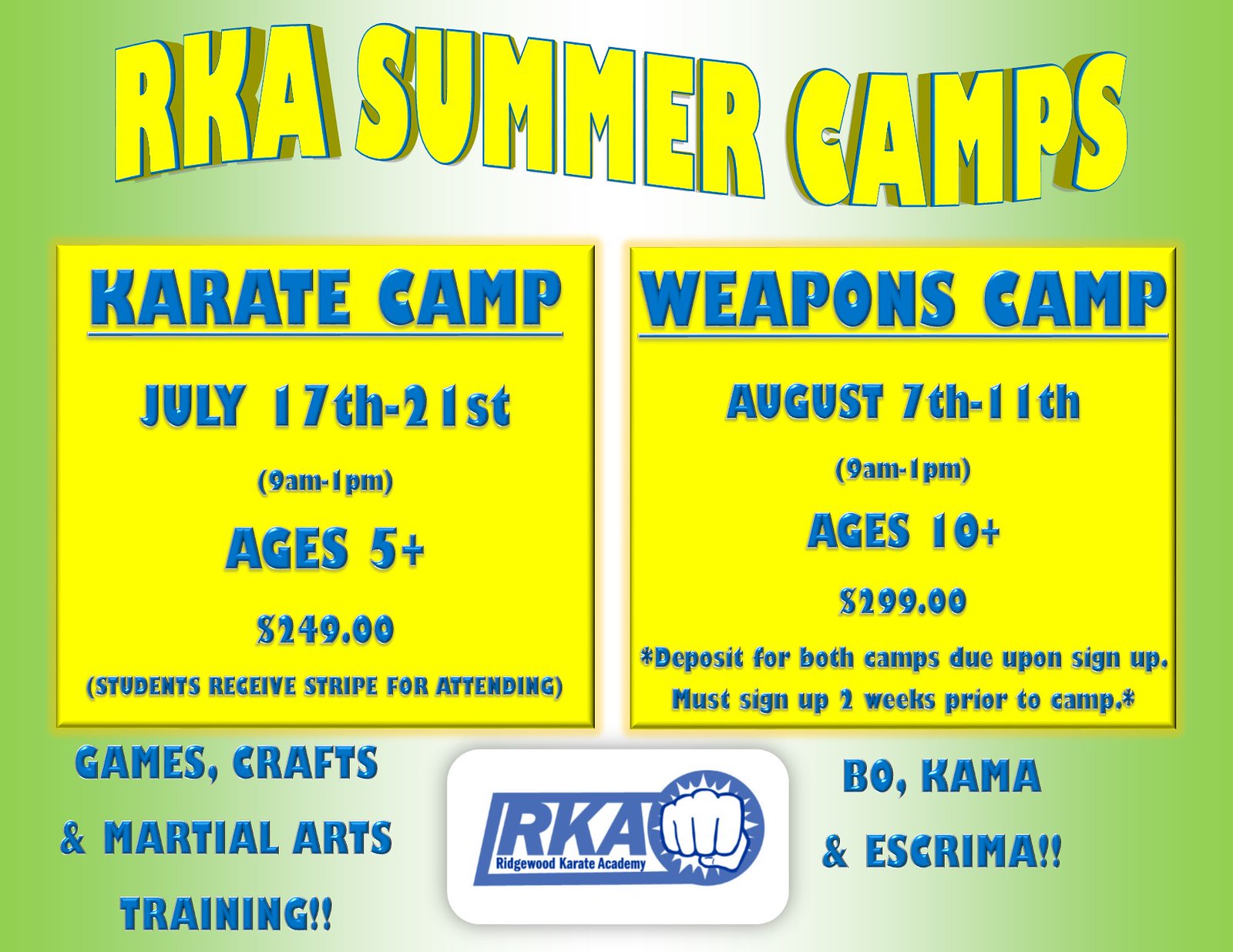The flyer for RKA Summer Camps features a vibrant green background that gradients to white towards the center. At the top, bold uppercase block letters declare "RKA SUMMER CAMPS." Below this header are two yellow squares with blue text, detailing the camp options. On the left, the Karate Camp is advertised, running from July 17th to the 21st, 9 a.m. to 1 p.m., for ages 5 and up at $249. Attending students receive a stripe. The right square promotes the Weapons Camp, scheduled for August 7th to the 11th, 9 a.m. to 1 p.m., for ages 10 and up at $299. Deposits for both camps are due upon sign-up and registration must be completed two weeks prior to each camp. The left side of the flyer, adorned with blue lettering, highlights activities such as games, crafts, and martial arts training. Centrally, a white rectangle features the RKA logo, a fist, and "RKA Ridgewood Karate Academy" in blue font, alongside the terms "Biokama and Eskrima." The overall design is eye-catching with its contrasting color scheme and structured layout, clearly presenting all the necessary information for prospective campers.